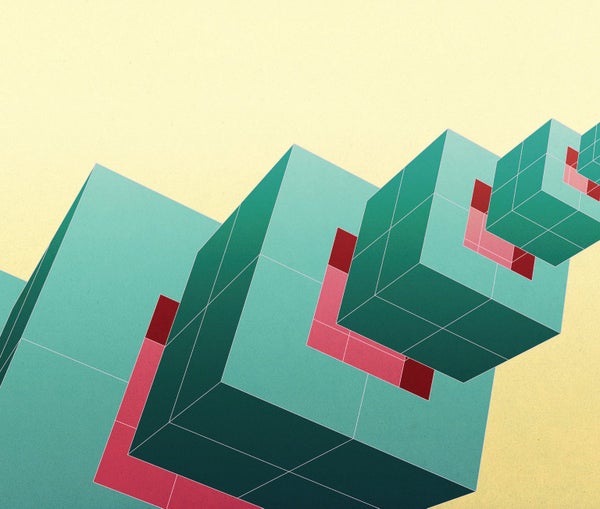The image features a visually striking, computer-generated scene containing a series of geometric cubes meticulously stacked and positioned in a diagonal arrangement from the lower left to the upper right. The cubes decrease in size as they ascend, creating a pyramid-like structure. The outer framework of these cubes is a distinct bluish-green hue, and each cube encompasses a vibrant center filled with squares that transition between shades of pink and red. The structural cubes are accentuated by prominent white lines, particularly observable on their sides. The entire composition is set against a solid cream or light peach background, complementing the abstract and cubist-inspired aesthetic. Overall, the piece combines elements of modern digital art with unique geometric abstraction.